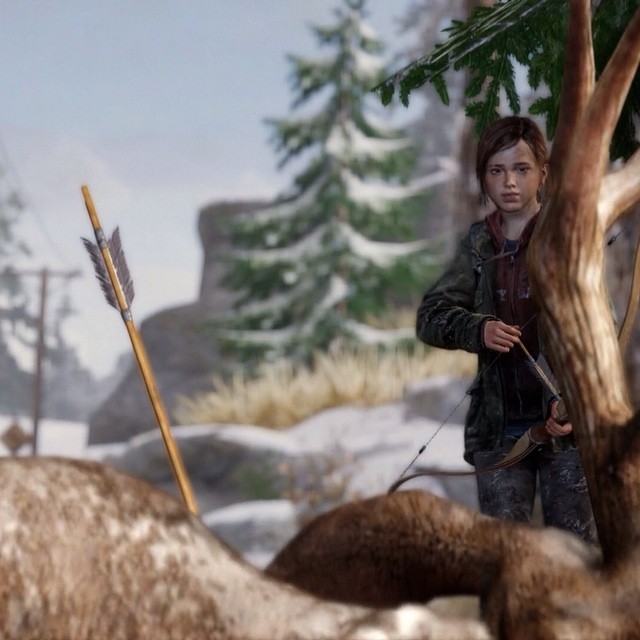In the digitally rendered image, a realistic yet subtly computer-generated scene unfolds. A girl is standing next to a tree in the background, her long hair intricately braided to the side of her head. She is poised with a bow and arrow in hand, gazing intently at an animal that appears to have been struck by one of her arrows. The arrow sticking out of the animal has beige feathered wing tips, adding a delicate detail to the scene. The animal itself is a mix of white and brown shades, suggesting it is likely a wild creature, with patches of dark brown fur. The snowy landscape adds a wintry chill, punctuated by the presence of a pine tree and a telephone pole with a sign in the distance, enhancing the sense of isolation and focus on the hunter and her prey.